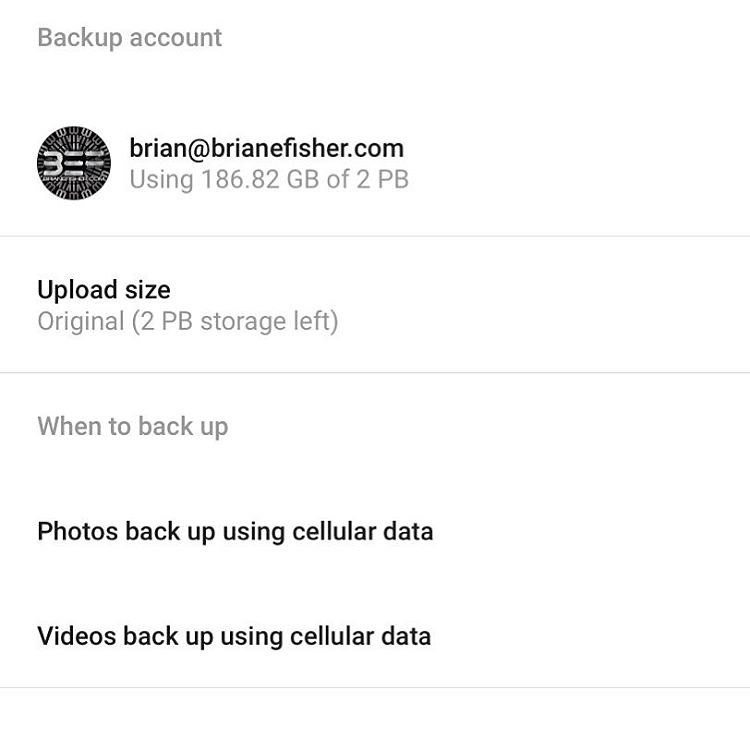The image showcases a user interface likely related to a backup account. At the very top, displayed in gray text, is the label "Backup Account." Directly beneath this label is a prominent, dark black circle featuring a silver number "3" inside it.

To the right of this circle, in bold black text, is the email address "brian@brianefisher.com." Underneath the email address, in lighter gray text, it is noted that the account is "Using 186.82 GB of 2PB."

Continuing downward, another piece of gray text indicates, "Upload size: Original," followed by a parenthetical note, "(2PB storage left)." A thin gray line spans the entire width of the white background area, creating a subtle separation.

Below the line, in a lighter shade of gray text, it states, "When to back up." About two inches below this text, in bold black letters, is the prompt "Photos back up using cellular data." 

Finally, another two inches lower, is the bold black text, "Videos back up using cellular data."

The overall background of this informational section is white, with the focal point being the dark black circle containing the silver number "3" and three adjacent silver lines, adding a slick, minimalist touch to the interface design.